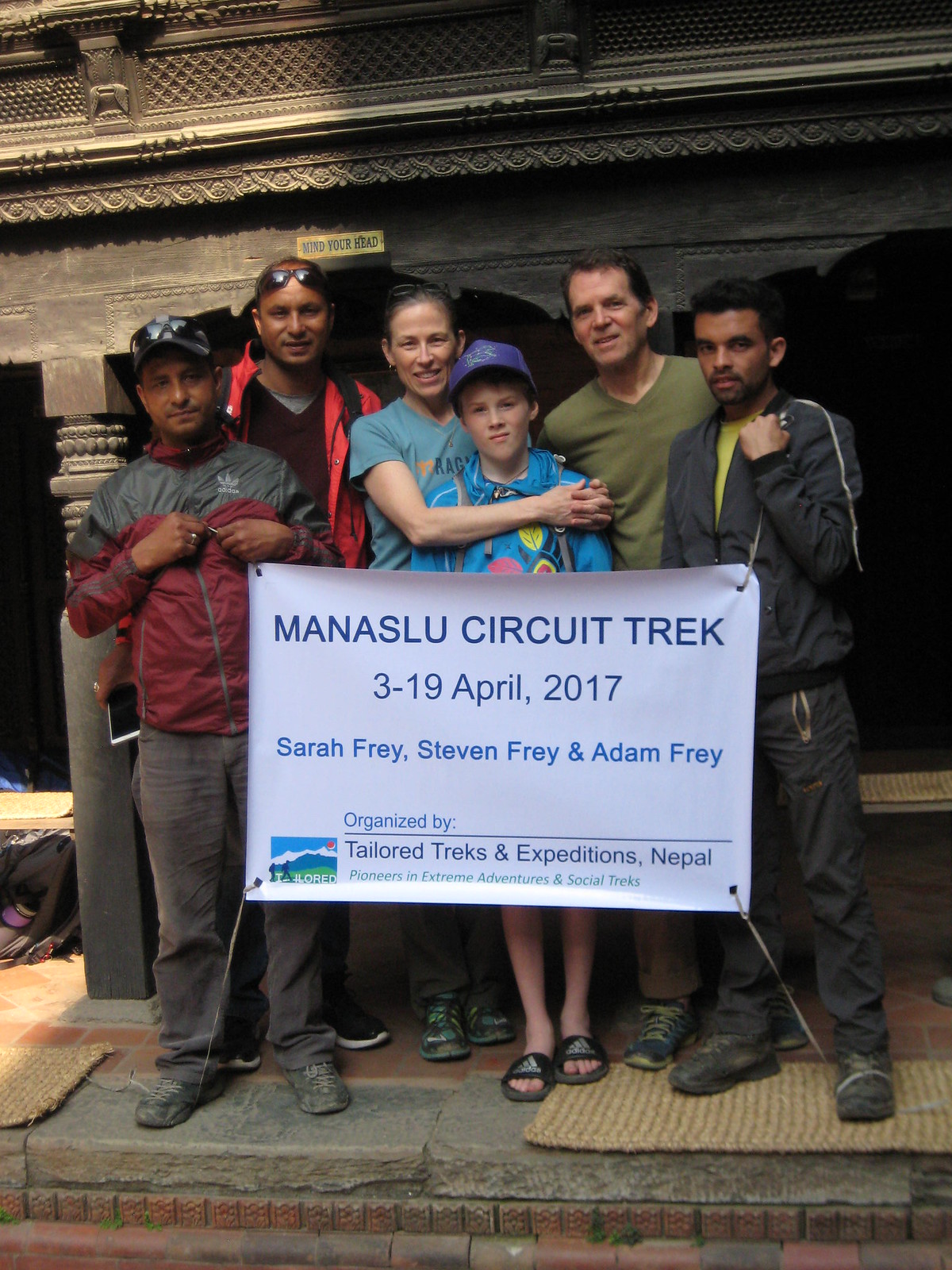The image features six people standing in front of a structure with gray pillars and an ornately designed facade and archways, evocative of an ancient or ceremonial building. They are positioned on a surface combining gray marble blocks and bricks, with one person standing on a woven ground rug. The central figures are the Frey family, comprising Sarah Frey, Stephen Frey, and Adam Frey. Sarah stands in the middle, her right arm wrapped around her son Adam, who sports a blue jacket, blue hat, bare legs, and sandals. Stephen is on Sarah's left, wearing a green V-neck shirt.

Adjacent to the Frey family are three members from the trekking group. On the left, one guide dons a purple and gray jacket with gray slacks and shoes, while behind him, another wears a purple shirt with sunglasses perched on his head and a robe draped over his left shoulder. To the right, a guide is clad in a gray jacket with a yellow shirt underneath, gray slacks with zippered pockets, and gray climbing boots.

They collectively hold a white banner with blue text that reads, "Manaslu Circuit Trek, April 3 to April 19, 2017," accompanied by the names Sarah Frey, Stephen Frey, and Adam Frey. The banner also notes that the trek was organized by Tailored Treks and Expeditions of Nepal, pioneers in extreme adventures and social treks. This photo appears to commemorate their successful expedition on the Manaslu Circuit Trek in April 2017.